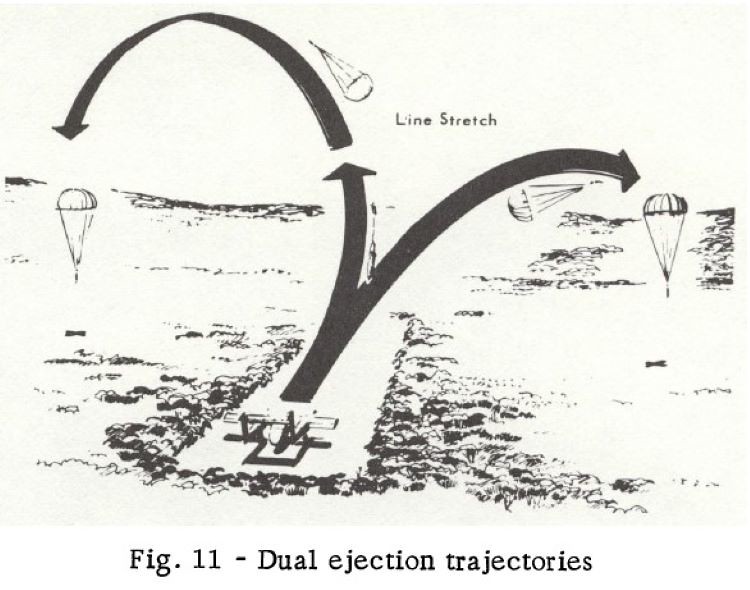The image is a detailed black-and-white drawing labeled at the bottom as "Figure 11 - Dual Ejection Trajectories." Centered in the illustration is a small drawn airplane positioned on what resembles a runway, flanked by depictions of earth or grass. From the front of the airplane, a thick black line ascends skyward before splitting into two distinct directions. 

To the right, the line continues, culminating in an arrow. Adjacent to this arrow are two parachutes: one depicted as coming down and the other veering off to the left. A similar thick black line extends to the left from the airplane, forming another arrow that briefly segments before resuming to the left, then curving downward. Another parachute is illustrated at the end of this pathway, with an additional parachute shown to the right of this final line. 

Within the intersection of these diverging lines, the text "Line Stretch" is indicated, emphasizing the point where the lines diverge. This intricate diagram visually represents the paths and outcomes associated with dual ejection trajectories.